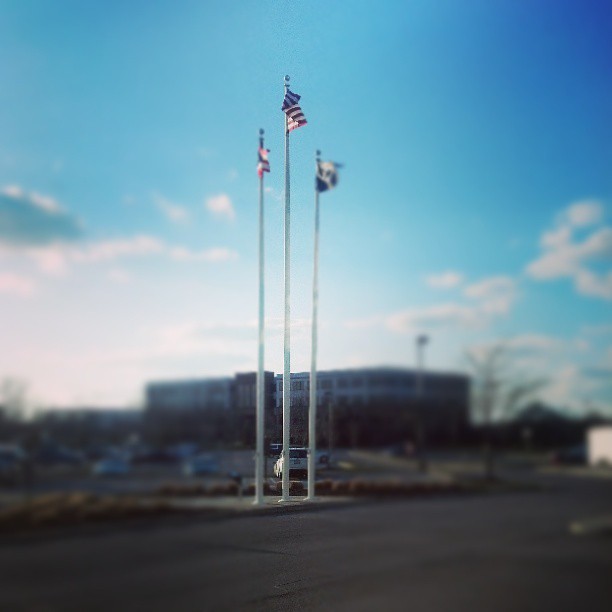This photograph captures three tall, white-painted flagpoles with flags fluttering at their tops. The central flag, prominently and clearly in focus, is the American flag, while the flags on either side are too blurred to discern, adding an element of mystery. The flagpoles are slightly staggered in height, with the American flag being the tallest. They are mounted on a slightly elevated grey concrete platform. The photographer has intentionally blurred the surroundings, emphasizing the flagpoles while a large building and a parking lot with a white SUV and other cars remain indistinct in the background. The image is set against a backdrop of a blue sky dotted with clouds, suggesting a clear day. Despite the poor editing, which makes the sharp-focus effect quite blatant, the photograph appears to aim for a symbolic representation, potentially highlighting national pride in an everyday setting.